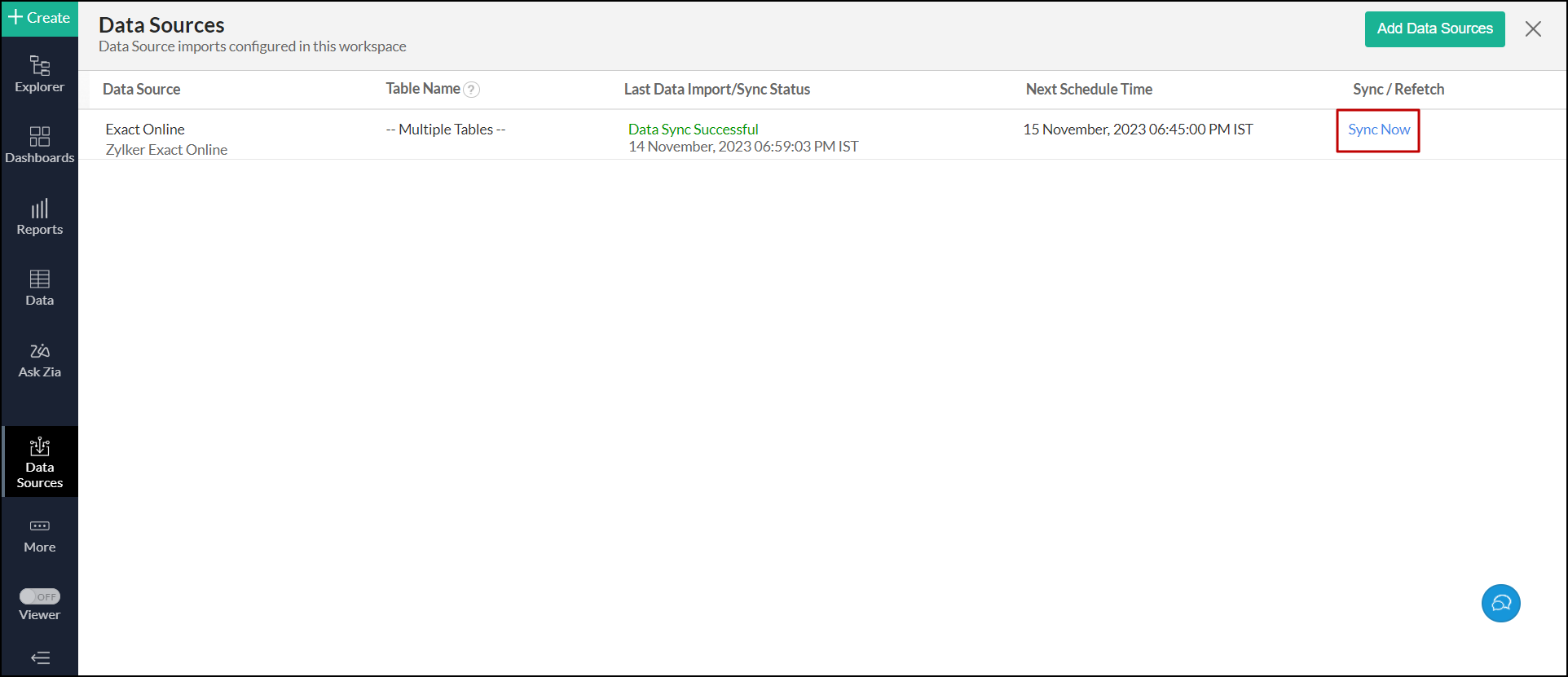The image is a detailed snapshot of a web page interface. 

In the top-left corner, there is a green box with a white plus sign and the word "CREATE" written in white. Right next to it, against a black background, it reads "Explore Dashboards" in white text. This section seems to outline the navigation options available to the user.

Across the top of the page, there is a gray-shaded horizontal bar with the words "Data Sources" in black. Below this header, it mentions: "Data Source Imports Configured in this Workspace."

In the top-right corner of the webpage, there's a green rectangle with the text "Add Data Source" in white. Adjacent to this button, in the far top-right, there is a small gray 'X' icon, likely used to close this section or notification.

The main background of the page is white, featuring a data table with the following headers: "Data Source," "Table Name," "Last Data Import/Sync Status," and "Next Scheduled Time Sync/Refetch." A gray line separates this header row from the content below.

Underneath the gray line, an entry displayed as "Exact Online Zyker Exact Online Multiple Tables" indicates a specific data source. Next to this, in green, it states "Data Sync Successful." Below this status, the next line shows two timestamps: "14 November 2023, 06:59:03 PM IST," representing the last data sync time, and "15 November 2023, 06:45 PM IST," indicating the next scheduled sync time.

On the far right of the row, there is a "Sync Now" option highlighted in blue text with a red box around it, allowing the user to manually trigger data synchronization.